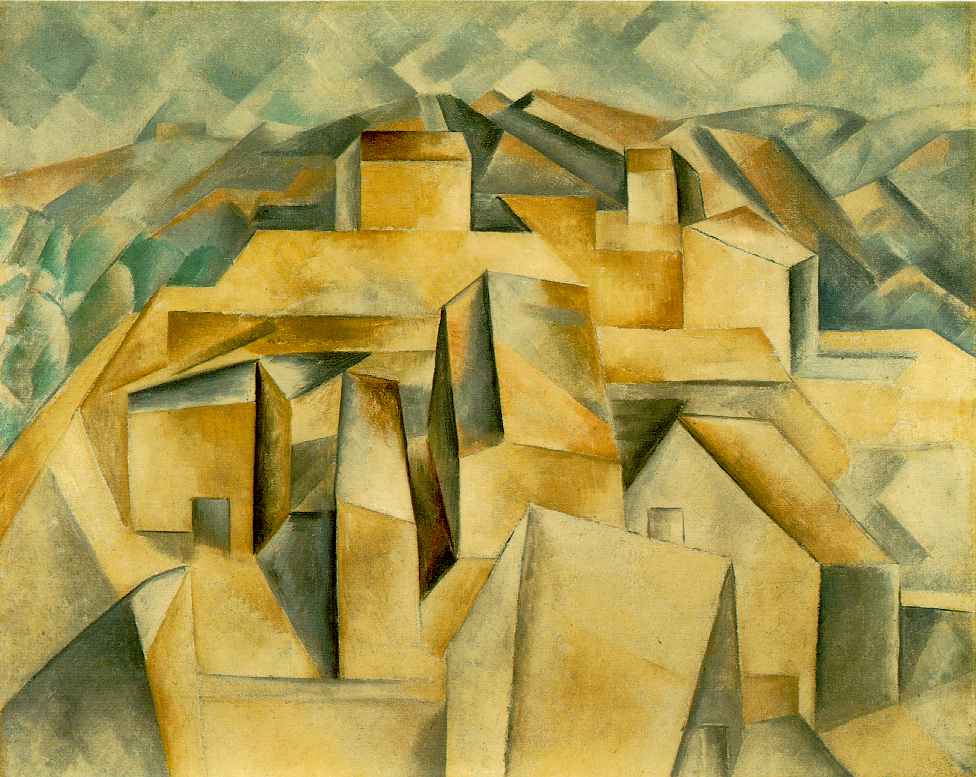This image is a landscape-oriented painting titled "Houses on a Hill," created by Pablo Picasso in 1909 in a cubism style. The painting, characterized by its modern abstract design, features a cityscape composed of angular, overlapping houses and structures. The dominant shapes are sharp angles, prisms, rectangles, and simple geometric forms. The color palette is primarily made up of tones of beige, brown, and aqua, with an orangish-brown used for most rooftops. In the background, there is a bluish-gray mountainscape and a sky painted in hash marks of light aqua and cream, adding to the overall angularity of the scene. The painting is devoid of any people, trees, or flowers, focusing solely on the rooftops and the background scenery, creating a symmetrical and visually striking composition.